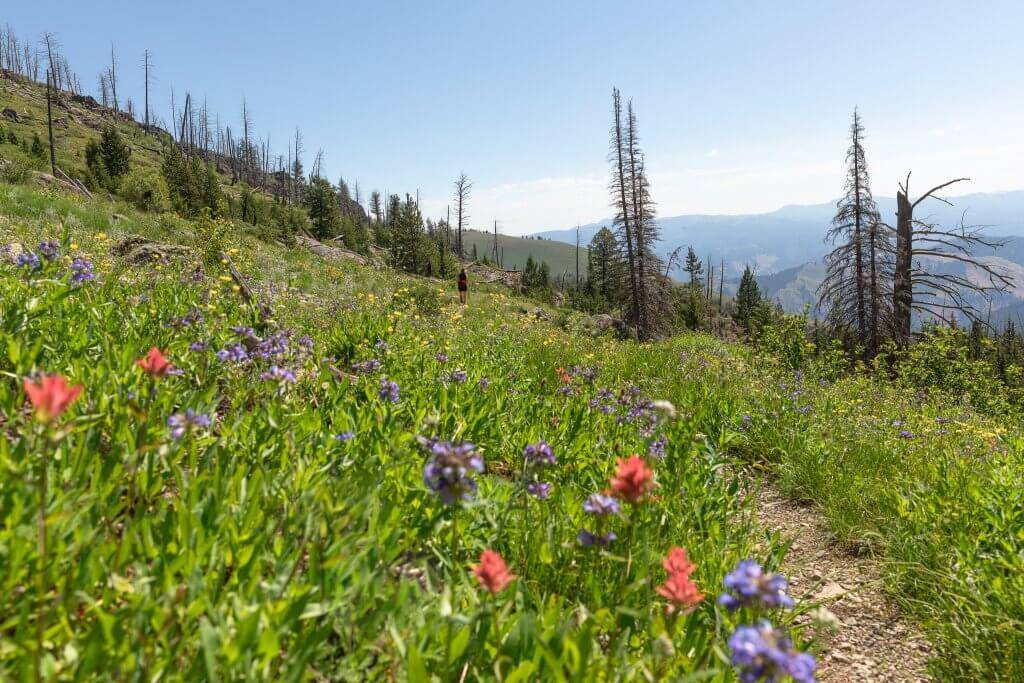The photograph captures a lush, detailed mountainside scene taken from a low perspective, close to the grass and flowers. It's a bright, sunny day, showcasing a vibrant, multi-colored array of wildflowers with pink, purple, red, yellow, and orange hues interspersed among green grasses. The path, worn from use, winds through this wild landscape and appears as a brown trail of dirt and leaves amidst the foliage. 

In the foreground, there are numerous trees, their branches bare and leafless, suggesting the advent of winter. One prominent tree stump catches the eye, broken and rugged. Further back, faint mountain ranges stretch across the horizon under a clear blue sky, dotted with white clouds. The mountains display a patchwork of greenery and open clearings, hinting at the varied terrain. 

A single figure, possibly a female, dressed in a red shirt and dark shorts, strides along the path, adding a touch of human presence to the tranquil natural setting. This solitary hiker in dark clothing is a distant yet integral part of the landscape, walking along the well-trodden path that meanders through the vibrant tapestry of flowers, wild grasses, and solemn, leafless trees.